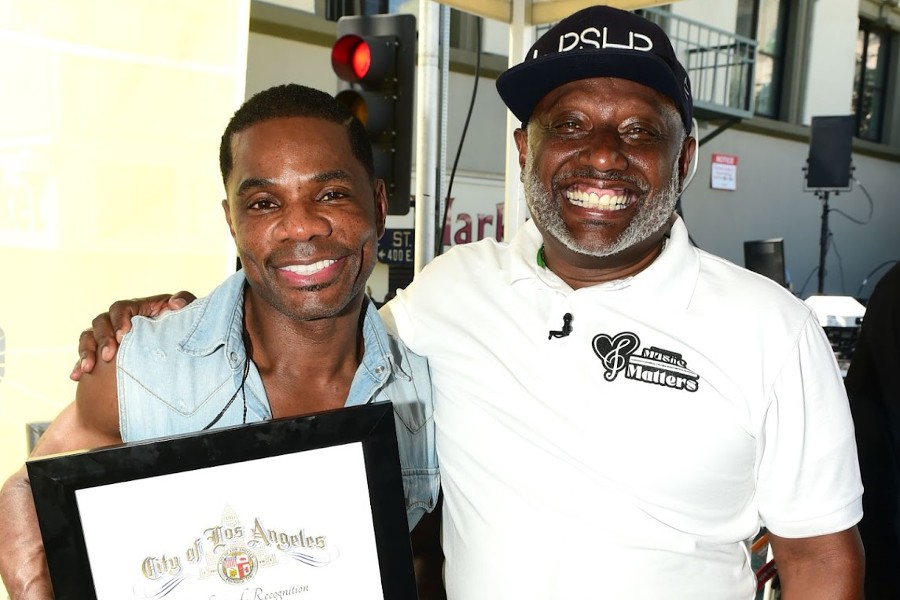In this image, two Black men stand side by side, both beaming with wide, genuine smiles. The man on the right is older, with a white beard and twinkling brown eyes. He dons a black cap with white text, a white T-shirt with the slogan "Music Matters," and a heart-shaped treble clef design. A microphone is clipped to his shirt, suggesting he's ready to address an audience or perform. His teeth are remarkably white, enhancing his cheerful expression.

Next to him on the left is a younger man with short black hair. He is wearing a sleeveless, open-neck jean vest and showcases his own bright smile, his wide nose adding to his distinguishing features. He holds an award from the City of Los Angeles, partially visible in a black frame, with the city's seal and the word "Recognition" prominently displayed.

The background hints at an outdoor setting with a red streetlight and a sign, possibly near a building. Monitors and other equipment are visible, suggesting some form of event or gathering is taking place, adding to the significance of their shared moment.